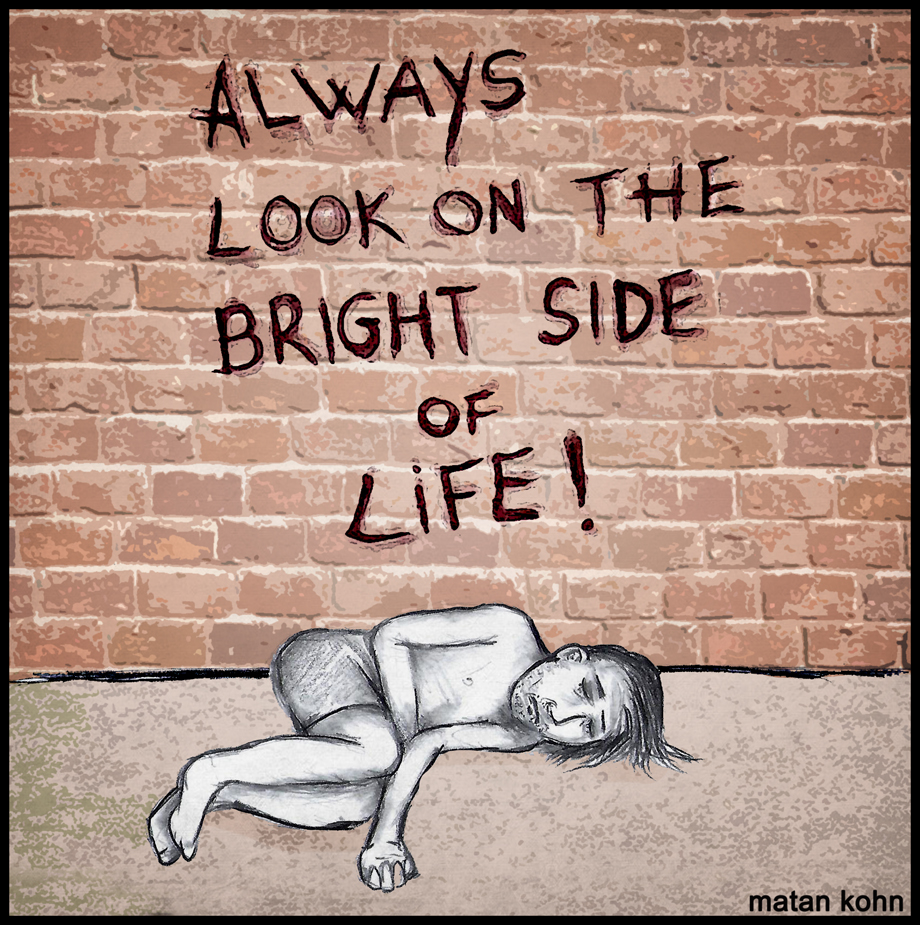The digital sketch depicts a somber scene with a striking contrast between its elements. At the center of the composition, a man is laying on a beige floor in front of a brick wall. The man is illustrated in black and white, devoid of color unlike the rest of the image. He is positioned on his left side in a half-fetal posture, with his right arm draped over his stomach, suggesting illness or discomfort. His face appears grimy and unwell, hinting at a possible state of distress, and his long hair touches the floor.

He is scantily clothed, wearing only a pair of shorts without any shirt or shoes, possibly indicating homelessness or drug addiction. On the brick wall behind him, a stark message written in what looks like blood-red ink reads, "Always look on the bright side of life!" followed by an exclamation point. The chilling and ironic tone of the message contrasts sharply with the man's condition. Additionally, the name "Matan Khan" is inscribed at the bottom right corner of the wall. A detail to note is a small patch of beige on the man's left hand, which could imply his involvement in the ominous writing on the wall.